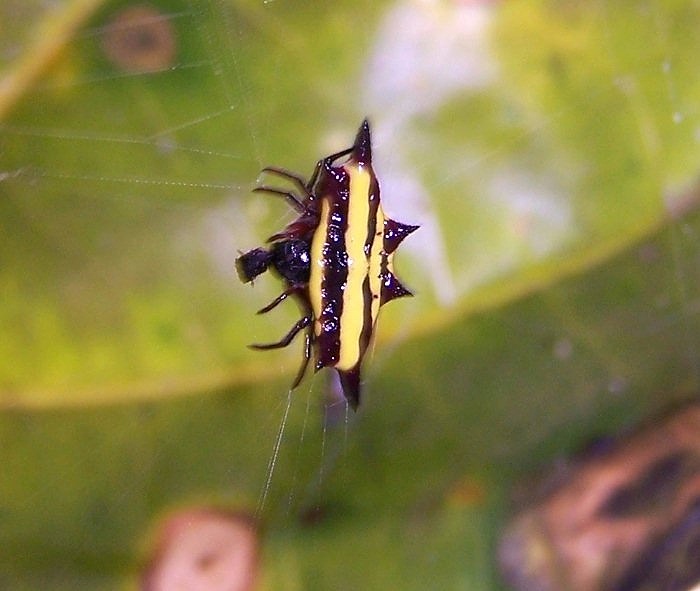This close-up, square photograph captures a peculiar insect suspended in a finely woven spider web, centered prominently in the frame. The insect, which resembles a small, crab-like beetle or possibly even a spider, has a glossy, almost slimy texture and features a mix of yellow and black stripes running across its body. It is adorned with small black spikes and exhibits no fewer than six visible legs. The creature also has two pointed horns protruding from the top of its head. The background, though blurred, reveals a large green leaf marked with visible veins and scattered brown spots, suggesting it's possibly a banana leaf in need of moisture. The insect's unusual appearance and the intricate details of the web and leaf create a fascinating but somewhat eerie image.